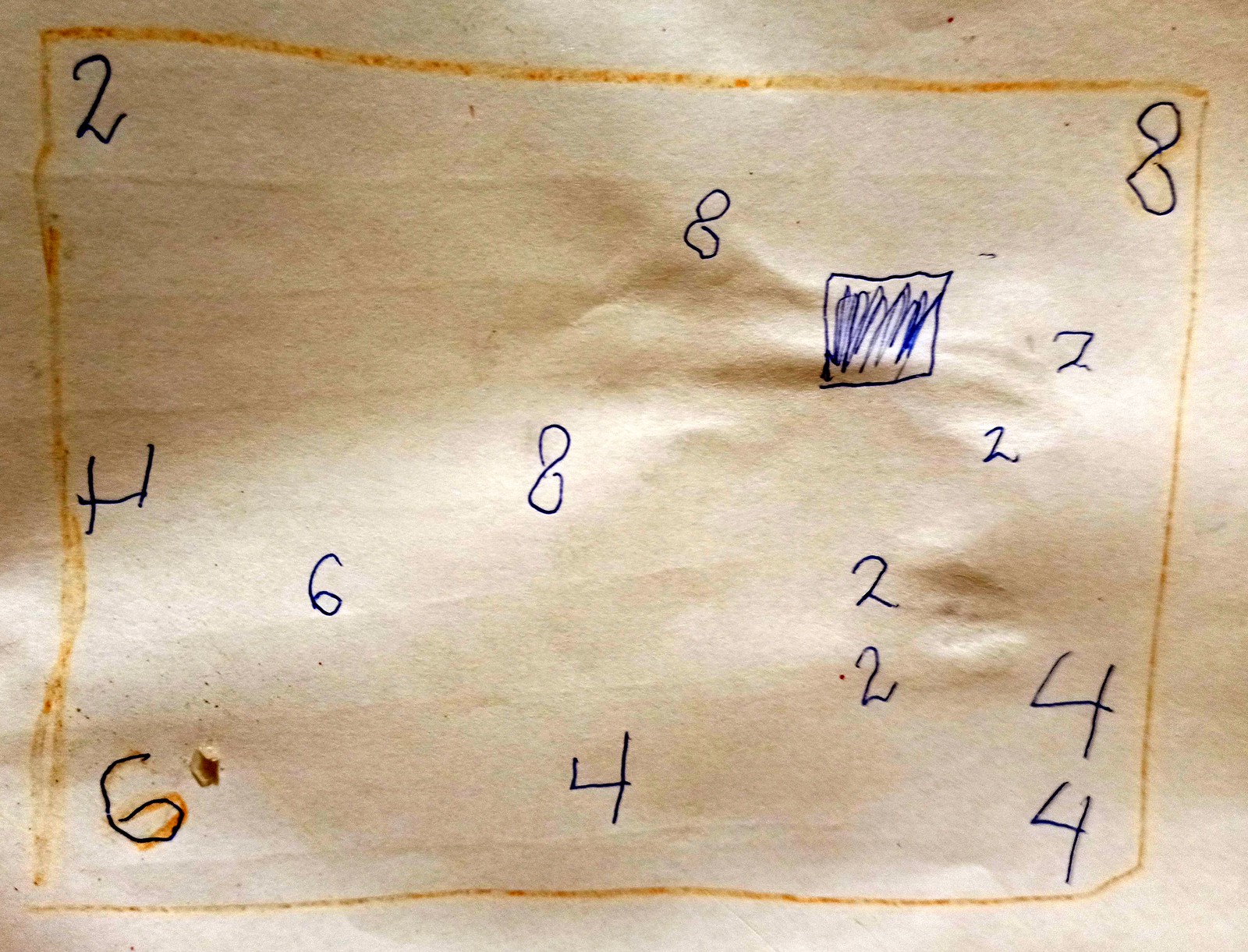This image displays a piece of white paper with varying shades of shadows across its surface. Dominating the center, there is a haphazardly drawn square box formed by a yellow crayon. The left vertical line of the box is notably curvy, while the right vertical line is perfectly straight. The bottom horizontal line exhibits a slight curve in the middle, contrasting with the more subtle sag in the middle of the top horizontal line.

Within and around this crayon box, various numbers are inscribed predominantly in blue ink, though some appear darker due to shadowing. In the top right corner of the crayon box, there is an '8' that appears black due to shadowing, but is originally blue. A blue '2' is located at the top left corner, while a backwards '4' marks the left vertical edge.

At the bottom of the box, a '6' is outlined in the same yellow crayon used to create the box. Near the bottom middle edge, there's another '4', along with a '4' situated at the bottom right corner, which has yet another '4' positioned directly above it. 

Additionally, the lower part of the crayon box features a vertical sequence of four '2's, stacked one atop the other. Above these, slightly to the right, are two more '2's positioned horizontally, one to the immediate left and below the upper ones. Furthermore, another inked box with intricate, squiggly lines inside can be found within the overall scene, enhancing the complexity of the composition.

This carefully detailed visual narrative captures the intricacies and whimsical nature of the hand-drawn annotations and markings on the paper.